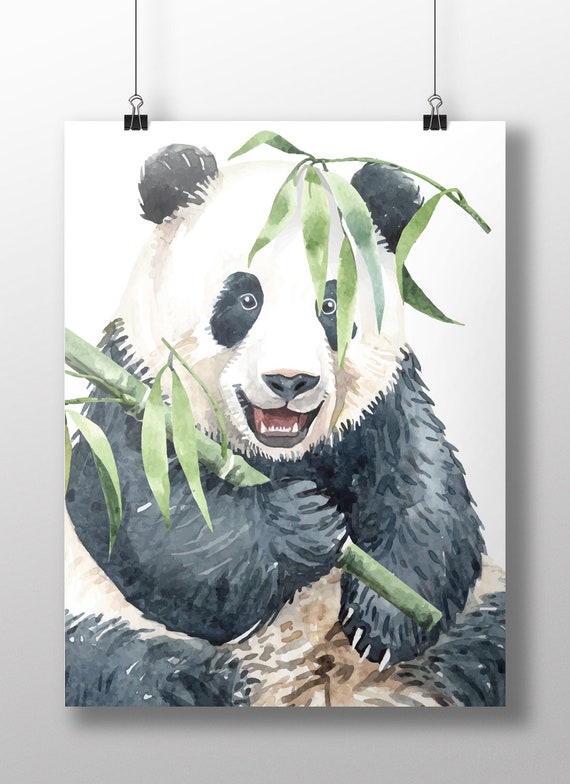The photograph captures a vibrant, computer-generated painting of a joyful panda on a white canvas paper. The panda, depicted in classic black and white with hints of red inside its mouth and a touch of tan on its lower belly, holds a bamboo stick with green leaves in its right paw. The panda's mouth is open in a big smile, showing large fangs that add a unique touch to the artwork. The panda looks straight ahead, with a branch of bamboo leaves amusingly placed on its head. This painting, with intricate details such as the panda's white claws and distinctive facial markings, is suspended by two black metal clips attached to black cords, creating a visually pleasing and well-lit display against a pale gray wall.